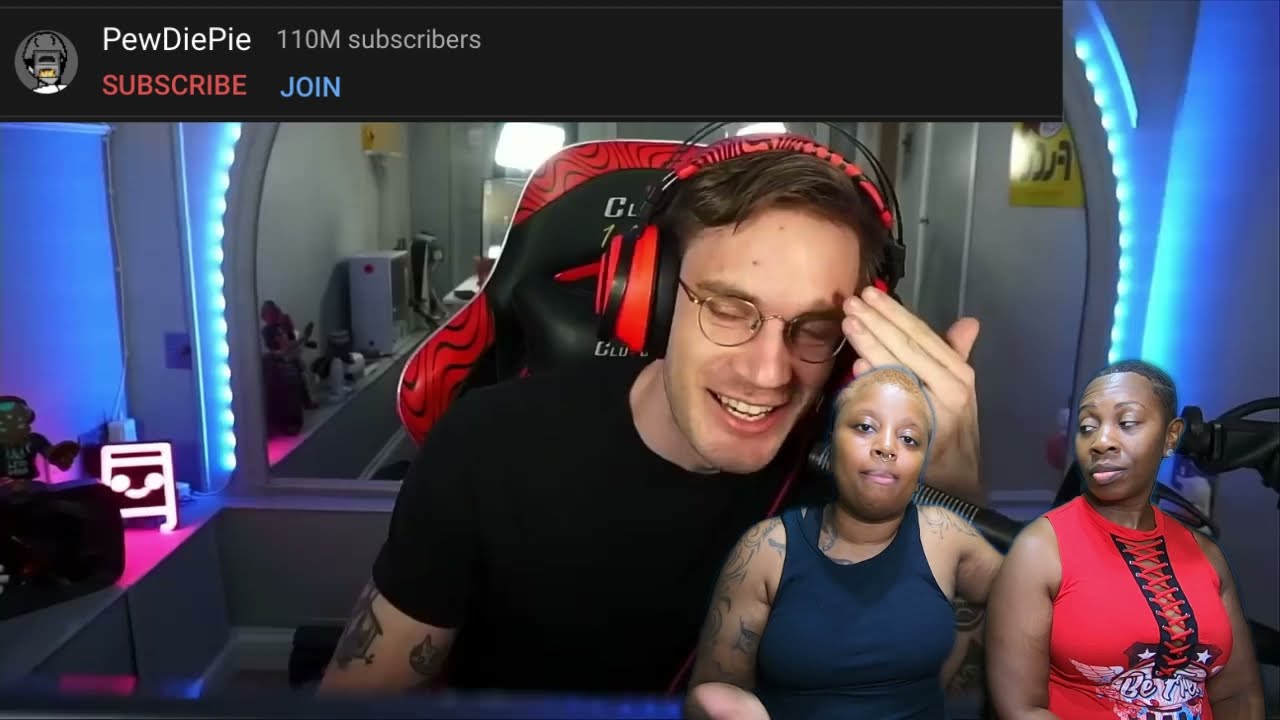In this image, a popular YouTuber, identified as PewDiePie with 110 million subscribers displayed in the upper left corner alongside options to subscribe and join, is the focal point. The image is horizontal and rectangular, placing PewDiePie—a young white man in his 20s or early 30s with short brown hair and dark gold to brown-rimmed glasses—prominently in the center. He is leaning slightly forward with his eyes closed and his hand touching his forehead, appearing deep in thought or possibly laughing. He wears a black t-shirt and a pair of red and black headphones that match his gaming chair, which features a red trim with black wave patterns.

Behind him, a mirror outlined with blue fluorescent lights casts a blue glow throughout the room, contributing to the ambient lighting. In the lower right-hand corner of the screen, there are two black women. The woman on the left, sporting a black tank top and tattoos, looks directly at the camera. The woman on the right, with short brown hair and a red sleeveless shirt featuring a netted design at the front, gazes at her companion. The scene suggests an active live stream or virtual interaction, possibly over a platform like Zoom.